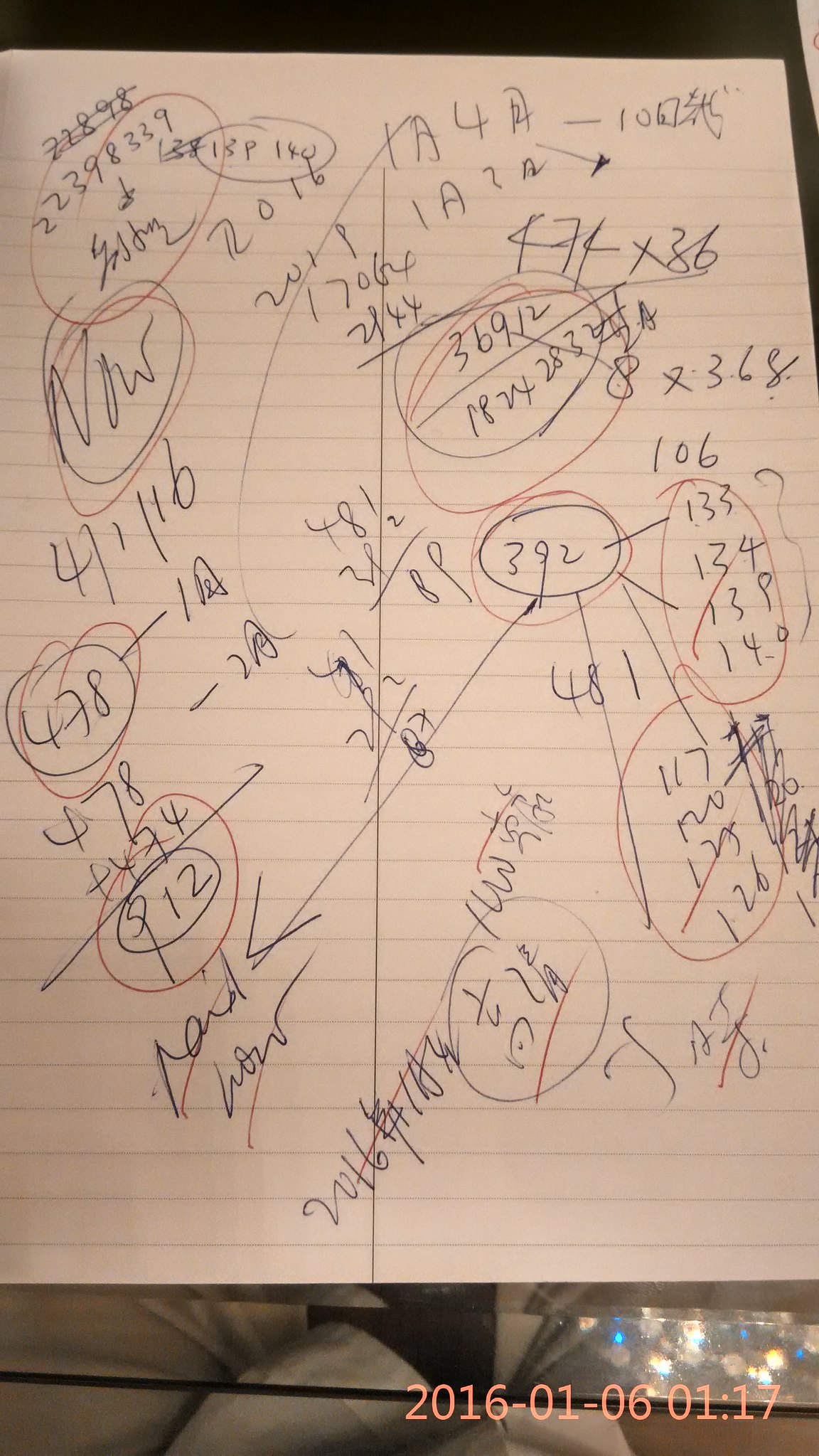The image features a sheet of paper adorned with horizontal lines reminiscent of those found in an exercise book or workbook. The paper is neatly divided into two halves by a vertically drawn line. Scattered across the sheet are numerous scribbles, primarily composed in black ink, indicating attempts at mathematical calculations. Visible among the black ink calculations are sums, divisions, and various numerical notations, alongside red ink circles highlighting specific numbers. This suggests a focused attempt at problem-solving or analysis. The paper itself rests on a glass surface, and in the lower right corner of the image, a time stamp and date stamp are clearly visible, adding a contextual temporal reference.